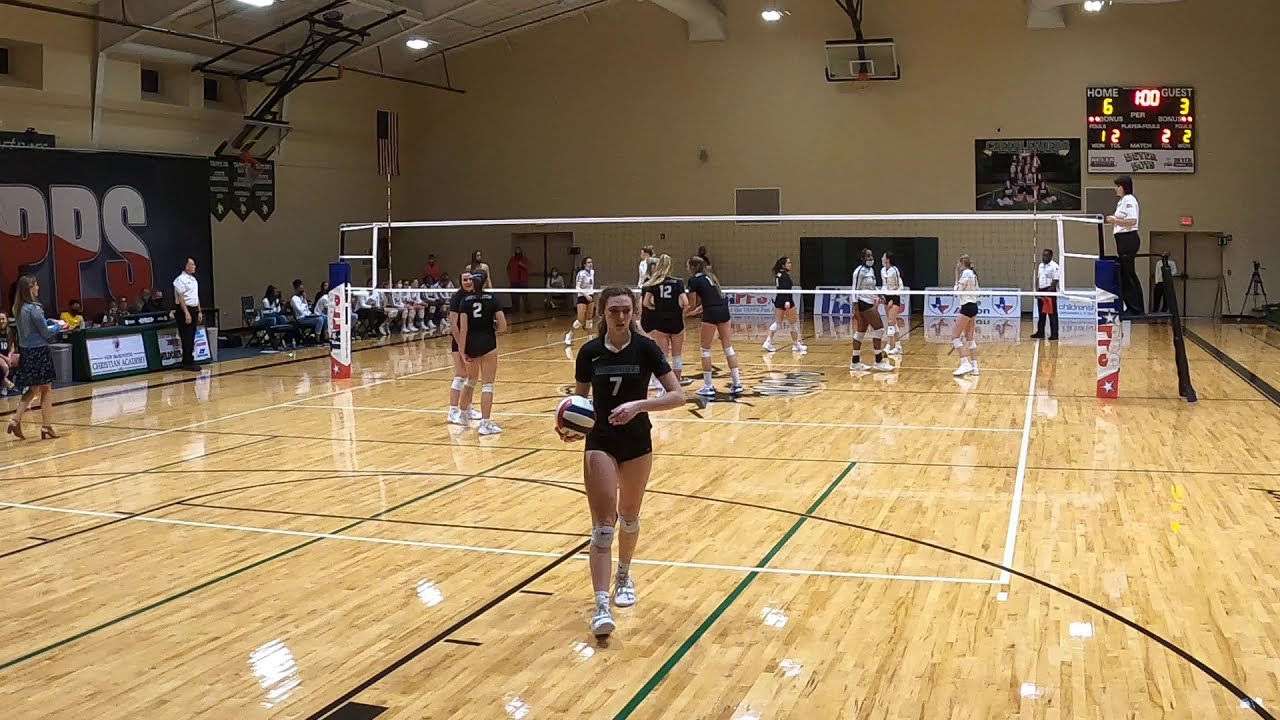In this detailed image of an indoor girls' volleyball match, the scene unfolds within what seems to be a high school gymnasium, evident from the raised basketball hoops leading to the ceiling. Prominently, at the center of the frame, stands a serious-faced teenage girl wearing a black uniform with the number 7. She is holding a volleyball and stepping away from her teammates, perhaps to retrieve another ball. The wooden floor beneath her feet has light brown hues with darker brown striations and is marked with lines for different sports, including a specific white line for volleyball.

The team in black uniforms with white tennis shoes occupies the front side of the image, while the opposing team in white jerseys and black shorts stands behind the white volleyball net that almost bisects the image. Both teams are preparing for or have just begun the match. A woman dressed in white and black is adjusting the net, indicating the game has yet to start. In the background, an adult can be seen walking across the court, and a black male is positioned at the far end.

On the left side of the court, a group of adults, possibly judges or officials, is seated at a table with a banner marked "PPS." Among them is a woman in a black skirt and light gray top, walking across in heels. The surroundings suggest activity and preparation, with various team members in the shot, including girls in uniforms numbered 2, 11, and 12.

The right side of the image showcases a scoreboard mounted on the wall that reads "Home 6, Guest 3," with illuminated dots beneath each score. At the center of the scoreboard, a timer indicating either 100 seconds or 1 minute is visible. A referee, standing atop a stand, overlooks the net, adding to the anticipatory atmosphere as the teams ready themselves for the match.